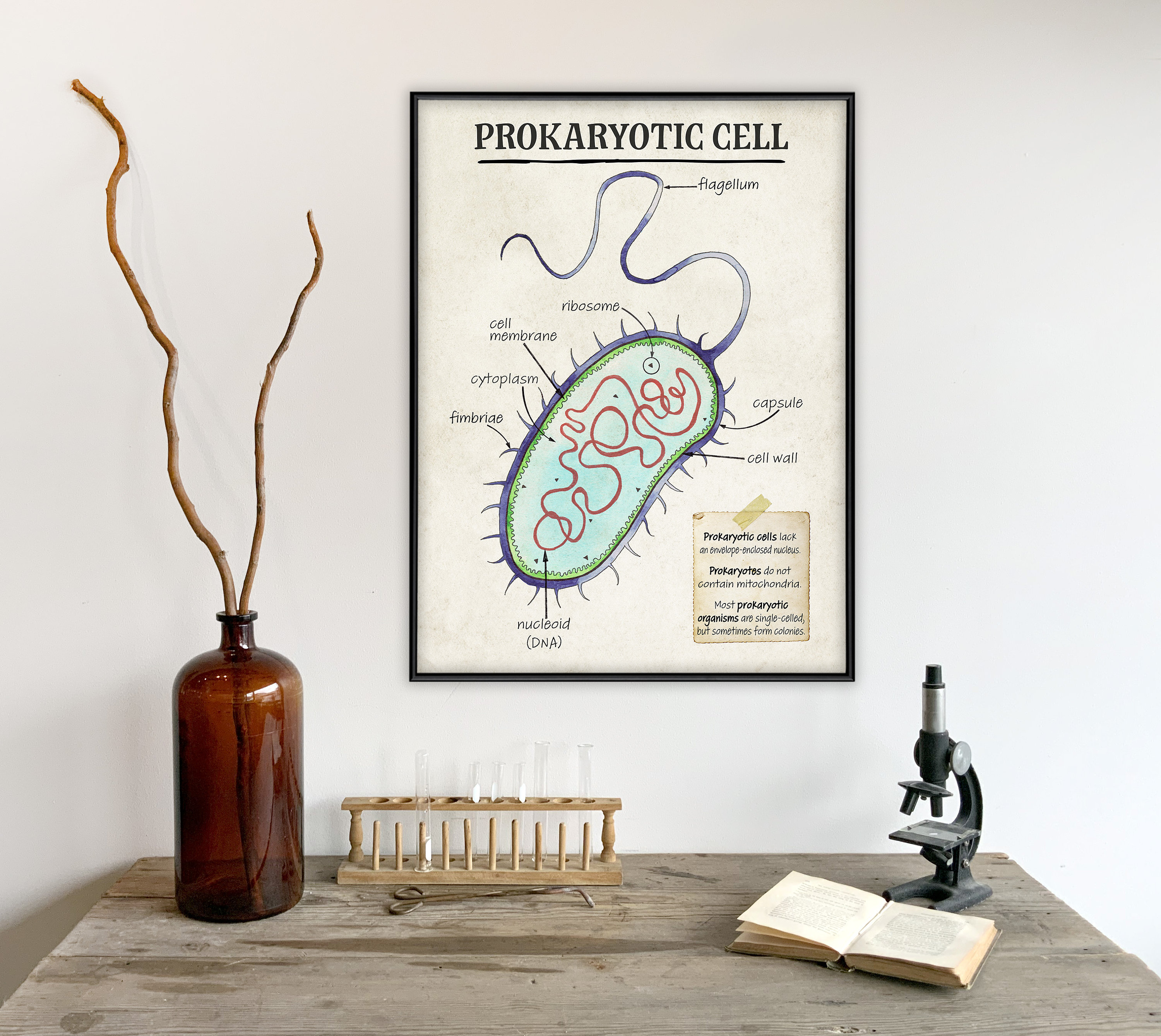This photograph depicts a rustic science lab setup centered around a table adorned with various scientific instruments. An open book lies at the table’s center, flanked by a sturdy microscope. Towards the back, a rack holds an array of test tubes. Dominating one side of the scene is a brown glass jug, reminiscent of old chemical containers, from which two long sticks protrude almost reaching the ceiling. Above the table, an educational poster illustrates a prokaryotic cell, complete with detailed labels for its components such as the flagellum, ribosome, cell membrane, cytoplasm, fimbriae, capsule, cell wall, and nucleoid. Text on a beige piece of paper affixed to the bottom right corner of the poster informs viewers that prokaryotic cells lack an envelope-enclosed nucleus and mitochondria, and though primarily single-celled, can sometimes form colonies. The backdrop is punctuated with hues of light blue, dark blue, purple, and various earth tones, providing a vintage, scholarly ambiance.